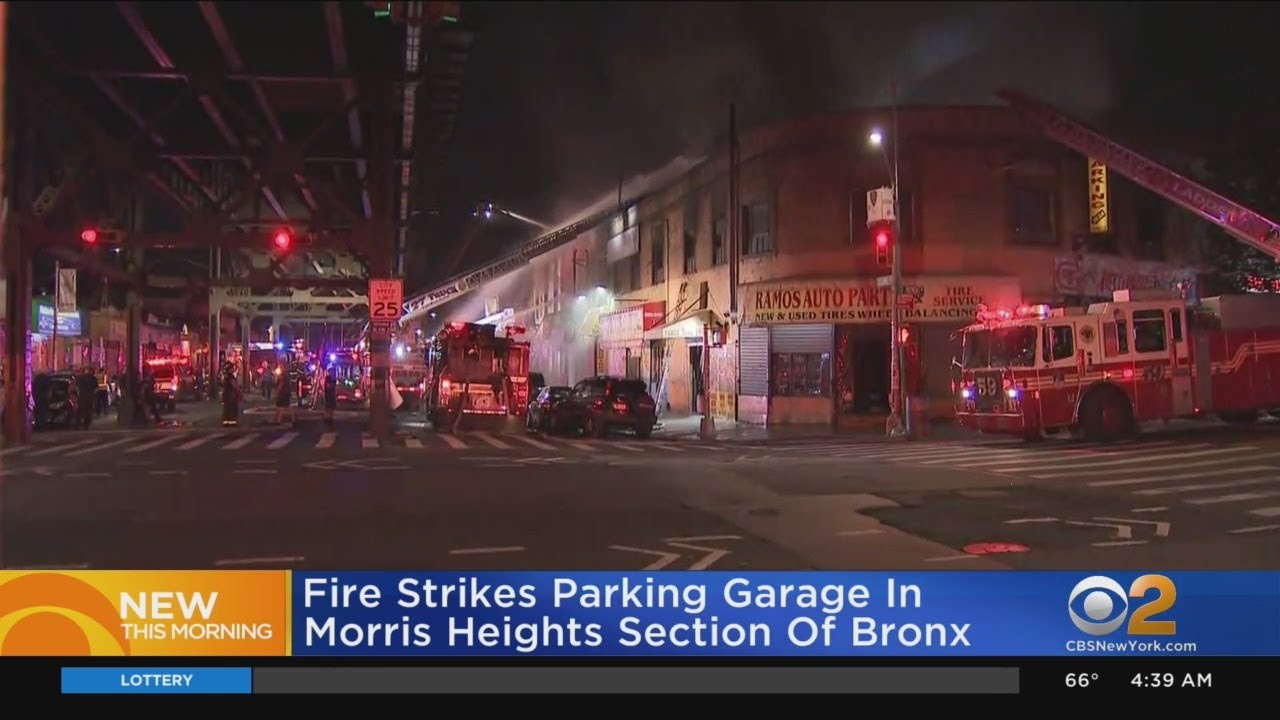The image is a detailed screenshot from a local TV broadcast reporting a fire in the Morris Heights section of the Bronx. The headline, displayed on an orange and blue banner with white text, reads, "New this morning, fire strikes parking garage in Morris Heights, section of the Bronx." The CBS News Network, CBSNewYork.com logo, and the number 2 are prominently featured next to the headline. The banner also includes information such as "66 degrees" and "4:39 AM" on the bottom right corner and the word "Lottery" on the bottom left.

In the scene, a fire truck is stationed on the right side, with its ladder extended towards the building. A group of people can be seen on the street as red emergency lights illuminate the area, casting a red tint over the surroundings. The location is characterized by a curved building and a string of connected old brick structures, typical of city blocks in New York. Additionally, there is a tall train bridge on the left-hand side running over the road. The fire truck appears to be actively addressing the fire, with a visible stream of water targeting the top of the building. The context and additional elements such as the possible entrance to a building labeled "Ramos Auto Parts" and the streetlight add depth to the scene, highlighting the urgency and scale of the emergency response.